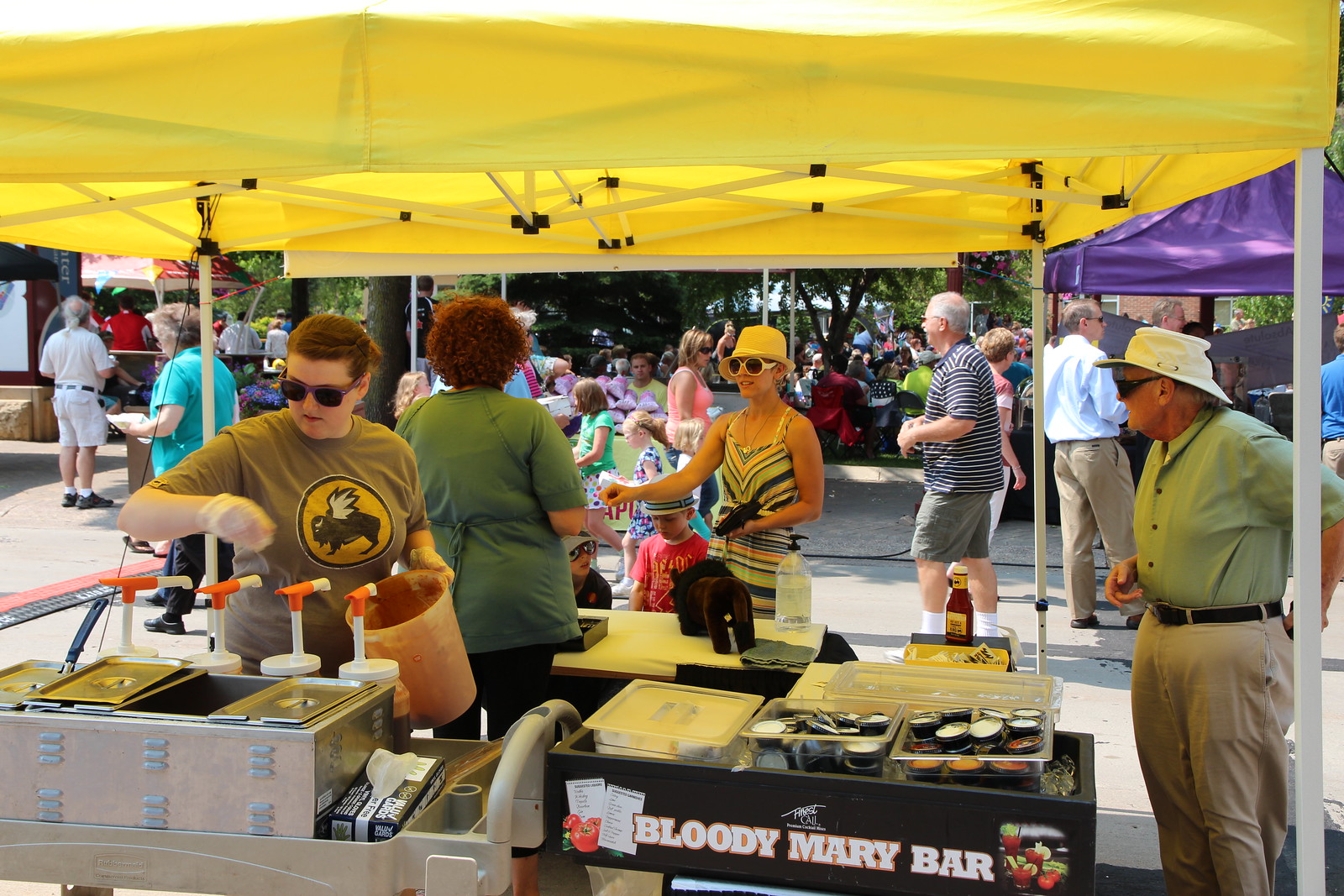The bustling outdoor scene captured in this photograph features a vibrant street fair teeming with activity. At the forefront is a portable tent with a distinct yellow canopy, its sides open to reveal two women preparing food. One woman, dressed in a gray shirt adorned with a winged buffalo emblem, stands near various cooking stations and abundant ramekins filled with different sauces. The signage on a black cooler inside the tent clearly reads "Bloody Mary Bar," highlighted by white font outlined in orange. Inside, another woman, clad in a green shirt and black pants, assists with the preparations. A woman wearing a yellow hat, white sunglasses, and a multicolored dress stands at the tent's counter, accompanied by her two small children—one in a red shirt—placing an order. Additional details include silver holders of vegetables and numerous pour bottles with white and orange handles scattered around. 

In the background, another cluster of people can be seen beneath a purple tent, indicating that the fair extends well beyond this one venue. The scene is dotted with canopies of various colors including blue, white, and red, supported by gleaming silver rods. On the far right, an older gentleman with gray hair, wearing a green shirt and tan pants, adds to the lively atmosphere along with a man in the background in a white and blue striped shirt and green shorts. The distant trees with their green leaves and brown trunks provide a leafy canopy, enhancing the festive and community-centered ambiance of this lively street fair.